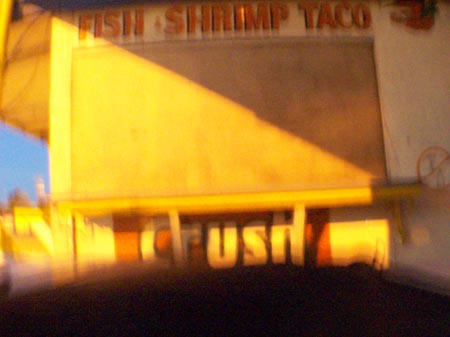A blurry photograph depicts a rundown takeout restaurant that appears to be closed. The scene is bathed in late afternoon sunlight, which reflects softly off the façade. The building's exterior is predominantly white, though it is in dire need of a fresh coat of paint. At the top of the structure, a pull-down shutter is firmly fastened, indicating the establishment is not currently in operation. Below the shutter is an ordering window, which is accompanied by a small counter supported by two wooden or similar types of brackets.

Directly above the ordering window, bold signage advertises "Fish, Shrimp, Taco" along with a small image that resembles either a taco or a palm tree on the beach. Beneath the counter, a red rectangular sign prominently displays the word "Crush" in white letters, each outlined in black. The setting suggests a once-bustling spot now standing still in its moment of respite.